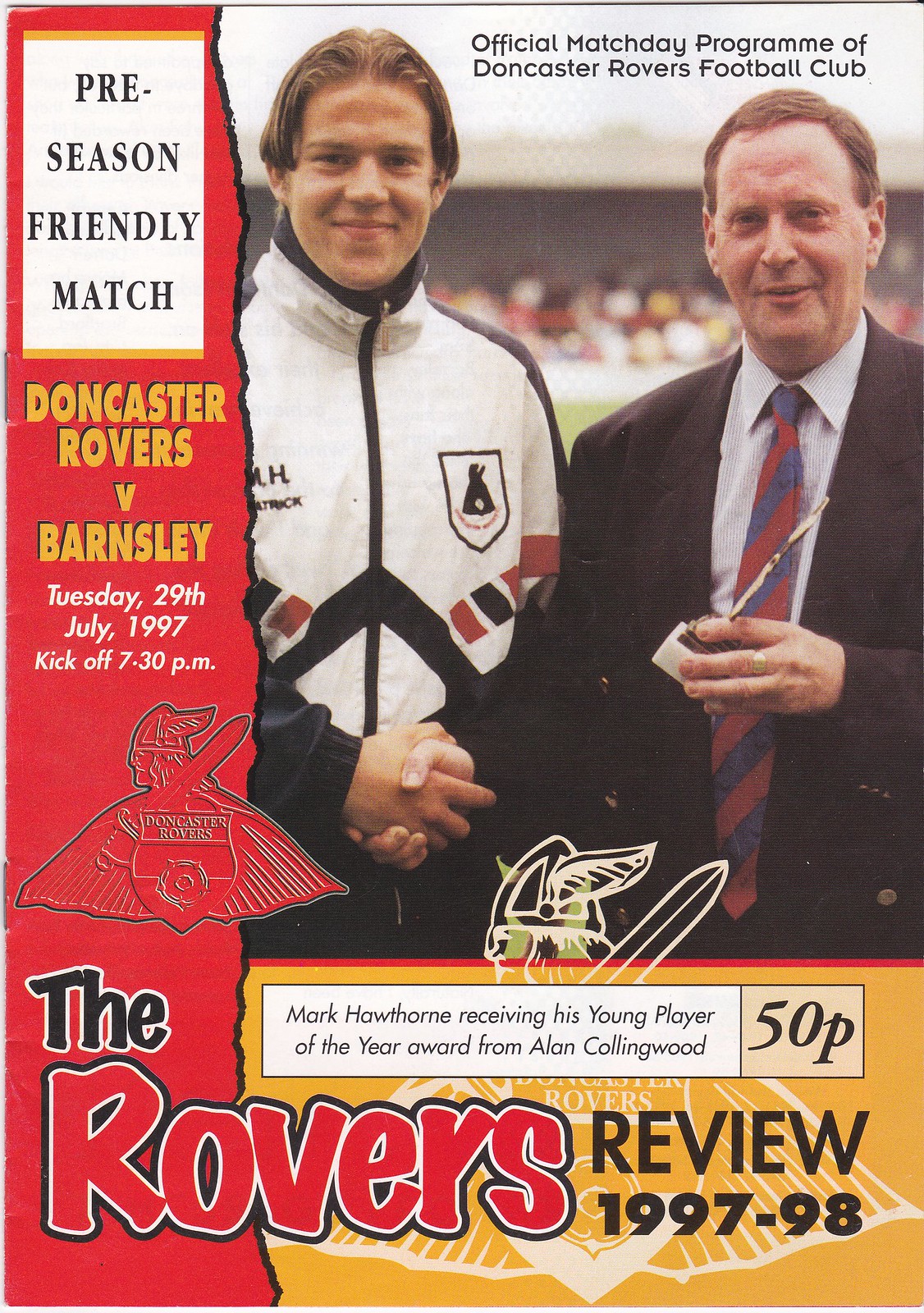The front cover of the 1997-1998 edition of "The Rover Review" magazine features a detailed and vibrant scene from a pre-season friendly match between Doncaster Rovers and Barnsley, held on Tuesday, July 29th, 1997, with a kickoff at 7:30 PM. Dominating the cover, Mark Hawthorne, the Young Player of the Year, is shown receiving his award from Alan Collingwood. Both men are engaged in a handshake; Hawthorne is dressed in a white sweat jacket with black and red accents, zipped up to the top, and featuring the team's symbol. Collingwood, in contrast, is clad in an unbuttoned black coat, a blue shirt, and a red-and-blue striped tie, holding the award in his right hand. The background showcases a blurred stadium filled with spectators. Below their hands, the team's mascot, resembling a Viking with a winged helmet and a shield, is prominently displayed alongside the club's crest. The title "The Rover's Review 1997-98" is printed in bold, mixed black and red font against a red backdrop on the left side of the cover, with additional details of the match in mustard yellow, black, and red text.